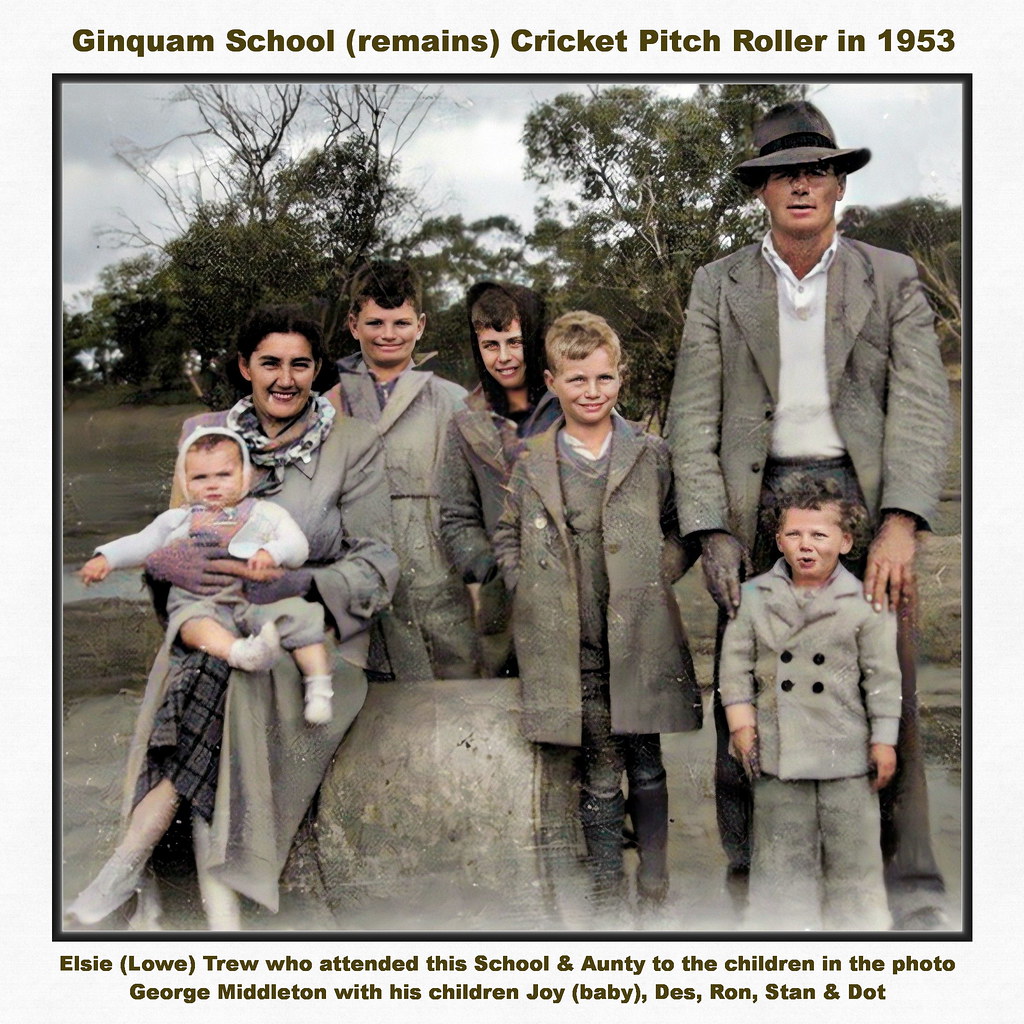The photograph from 1953, titled "Ginquam School Remains (Cricket Pitch Roller)," shows a multigenerational family posed together. The image, featuring noticeable dust and scratches indicative of its age, is in color but of low quality, suggesting an analog origin. Seven individuals are present, ranging in age, and likely comprise a single family. On the left, an infant wearing a bonnet or cap, a light gray jacket, and light gray pants is seated on the lap of its mother, who dons a checked or plaid dress in black and gray hues. The father, George Middleton, stands to the far right, distinguished by his darker or almost black right hand. In front of him stands a small boy in a light jacket. Others in the photograph include Auntie Elsie Lowe, who attended Ginquam School, and Middleton's children: Joy (the baby), Des, Ron, Stan, and Dot, spanning from approximately 5 to 12 years old.